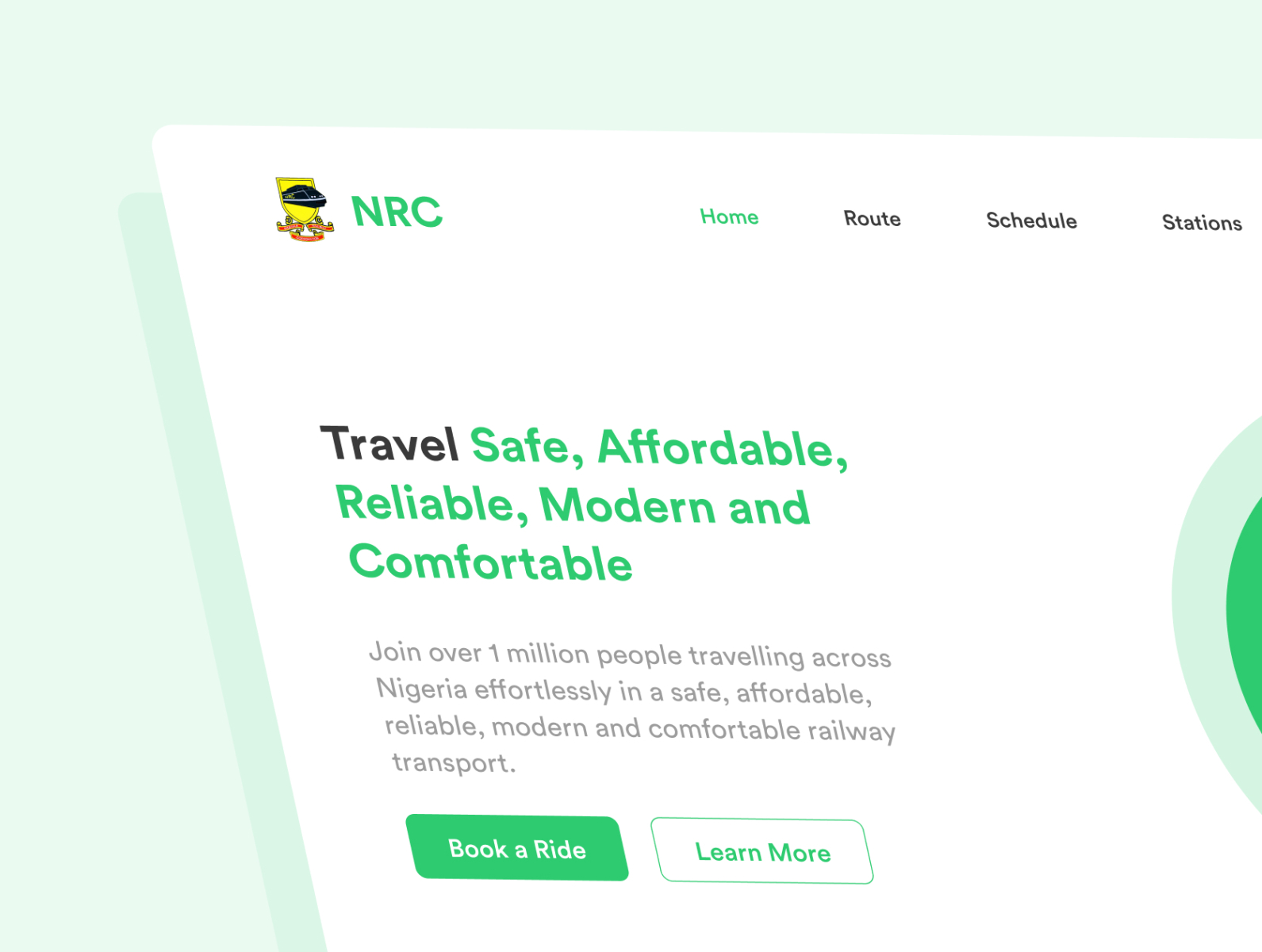This image appears slightly distorted, with the top portion leaning further left compared to the bottom. At the top, a prominent yellow symbol alongside the abbreviation "NRC" is displayed. Across the top row of the webpage, there are navigation tabs labeled "Home" in blue, "Route," "Schedule," and "Stations." 

On the left side, a bold heading reads "Travel Safe, Affordable, Reliable, Modern, and Comfortable." Below this header, light text invites users to "Join over one million people traveling across Nigeria effortlessly in a safe, affordable, reliable, modern, and comfortable railway transport."

Beneath this text, there are two clickable buttons: a green button labeled "Book a Ride" and a white button with blue text that says "Learn More."

On the right side of the page, a large circular design is partially visible due to the page cutoff. The outer edge of this circle is light blue, and it transitions to a dark green color in the middle. The overall composition appears to focus on promoting NRC's railway services in Nigeria, emphasizing convenience and safety.